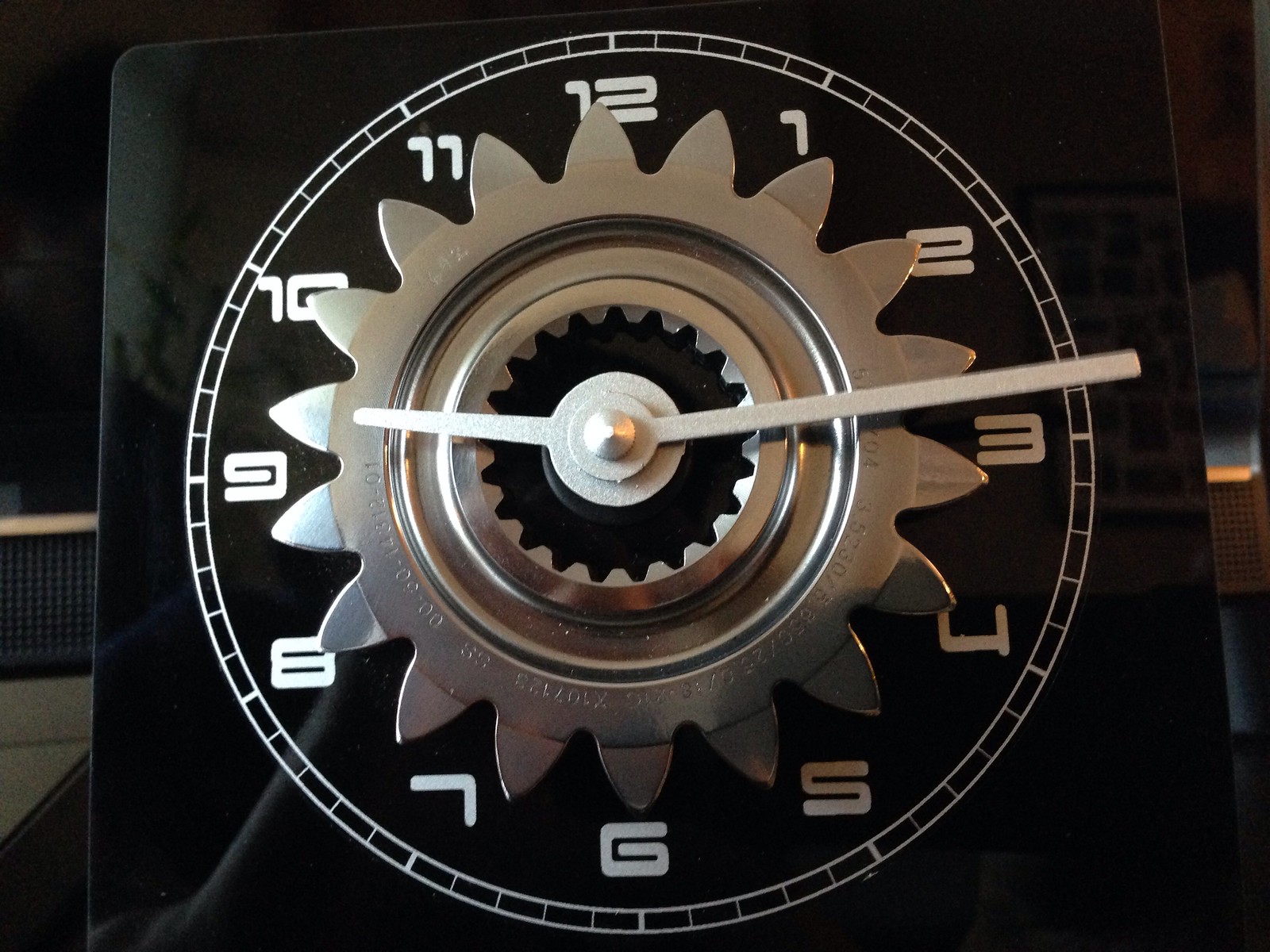The image showcases a uniquely designed clock with an eye-catching dark glass background, which is reflective enough to capture faint images of a wall and the person taking the photograph. At the center of the clock is a striking silver gear, intricately detailed and reminiscent of a sunflower with its layered, petal-like structure. Surrounding this central gear are two concentric white circles that demarcate the clock's face. The numbers 1 through 12 are evenly spaced around the perimeter, arranged in the customary clockwise fashion. Central to the design, within the innermost white circle, are two silvery clock hands that delicately point to the current time. Based on the position of the clock hands, the image was captured at approximately 9:13.